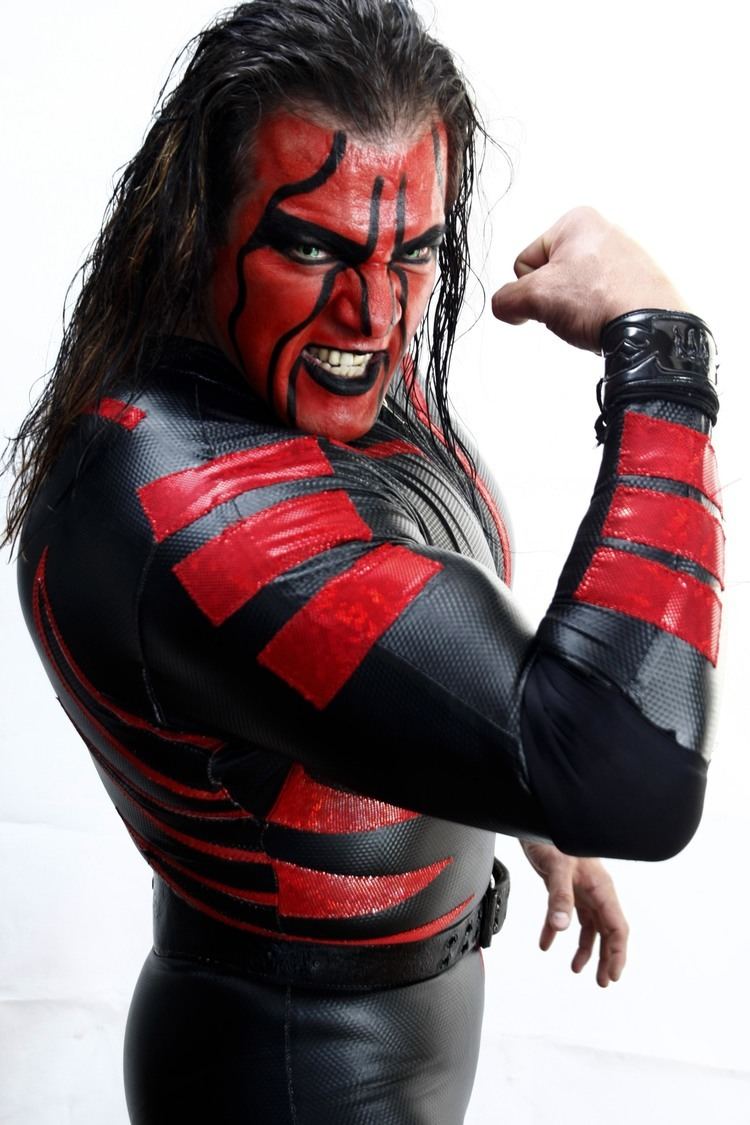The image depicts a Caucasian man in what appears to be a professional wrestler or superhero outfit, set against a white background. He is wearing a tight, black leather jumpsuit with a black belt and black pants. The suit features multiple red duct tape-like stripes: three on each shoulder, three on each forearm, and several across the chest, waist, and back. The man is facing his body to the right, flexing his right bicep with a clenched fist, showcasing the muscle. His head is turned towards the viewer with a growl on his face, showing his teeth as if in a menacing expression. His long, dark brown hair flows past his shoulders. His face is vividly painted red with intricate black stripes running from his forehead to his nose, around his eyes, and with a thick black outline around his eyes, giving a devil-like appearance. He may even be wearing special contact lenses to enhance his intense look.